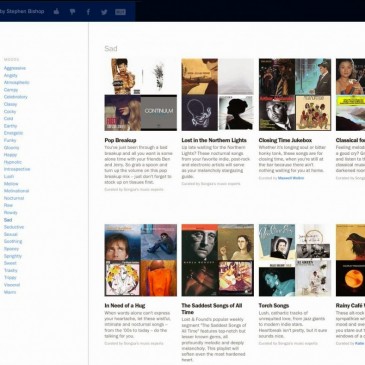The image depicts a webpage with a user interface featuring several distinct elements. At the top left corner, there are numerous tabs set against a blue background, clearly labeled "Tabs." Adjacent to these tabs, social media icons for Like, Dislike, Facebook, and Twitter are prominently displayed.

On the left side of the webpage, there is a vertical menu presented in a list format, also set in blue. The page's main content area, however, appears blurry and is not easily discernible. 

On the right side of the page, a series of articles are arranged vertically. Above this section, a header reads "Said." The first article is titled "Pop, Pick Up," followed by "Lost in the Northern Light." Subsequent articles include "Closing Time, Out of Box," "In the Need of a Pick," and "The Saddest Soaps of All Time, Trending Songs." These titles are written in black text against a white background.

Each article is accompanied by images, although the overall image quality is grainy, making the pictures' details unclear. The images themselves vary in color, including blue, black, and yellow tones.